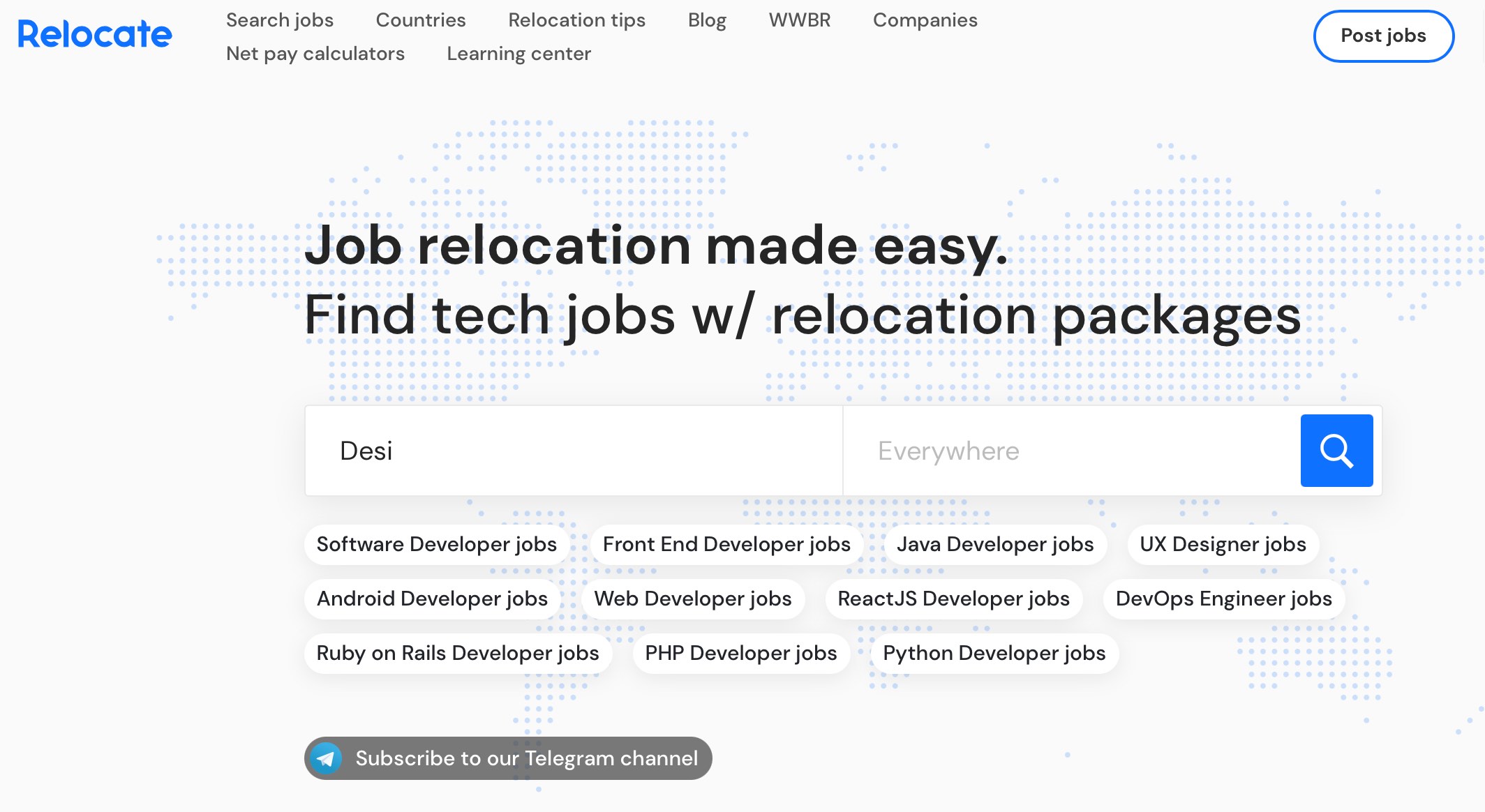This image is a section of the Relocate website. The background is an off-white shade, almost white but with a subtle difference. The company's name, "Relocate," is prominently displayed in a striking shade of blue reminiscent of Microsoft's branding. At the top of the page, a gray navigation menu allows users to search for jobs, explore different countries, access relocation tips, read the blog, and utilize features like WWBR, companies, NetPay Calculator, and Learning Center. Towards the far right, there are options to print the page in black text and a white button bordered in blue that says "Post Jobs".

Below the navigation menu, there is a subtle map serving as the background. This map is composed of tiny, light blue squares that give it a dot matrix-like appearance, portraying a flattened globe. Overlaid on the map, in bold font, is the headline "Job Relocation Made Easy." Directly below, a subheading reads, "Find Tech Jobs With Relocation Packages." Beneath this text, there is a search bar with the keyword "DESI" pre-entered, and a small magnifying glass icon to initiate the search for tech jobs near DESI.